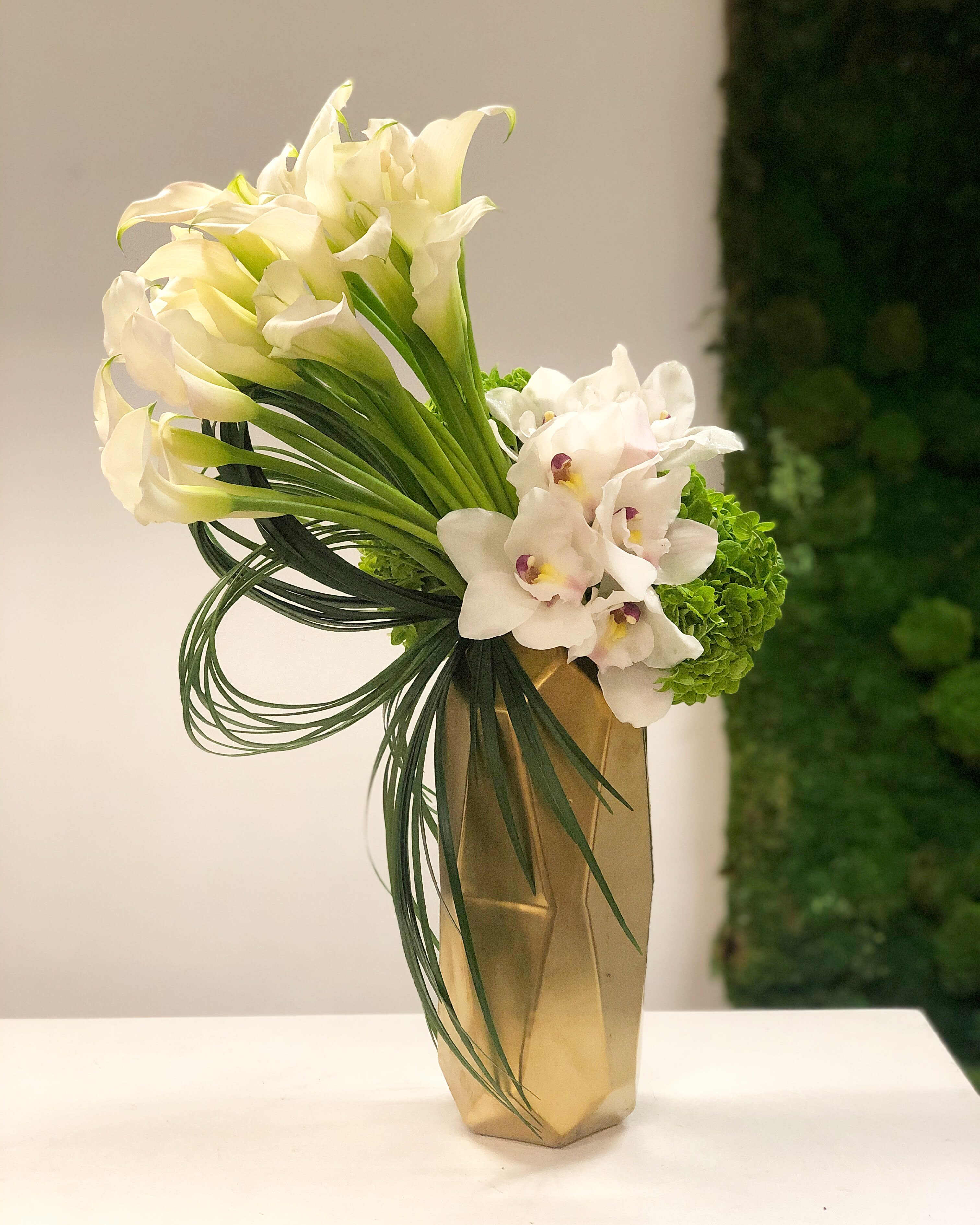A golden oblong vase, embellished with geometric jagged edges and seemingly made of a gold-colored plastic, stands on a white tabletop. The vase is brimming with a vibrant floral arrangement, prominently featuring around 13-15 elegant Calla Lilies with white petals. Alongside them are white daffodils, each revealing a distinct purple-brown interior deep within the bloom. Accompanying the flowers is a lush assortment of green leaves, and a green ribbon that appears to be tied into a bow, harmonizing with the foliage. The background consists of a white wall to the left and a section on the right adorned with a rich tapestry of green leaves, creating a blend of varying shades of green as they catch the light.